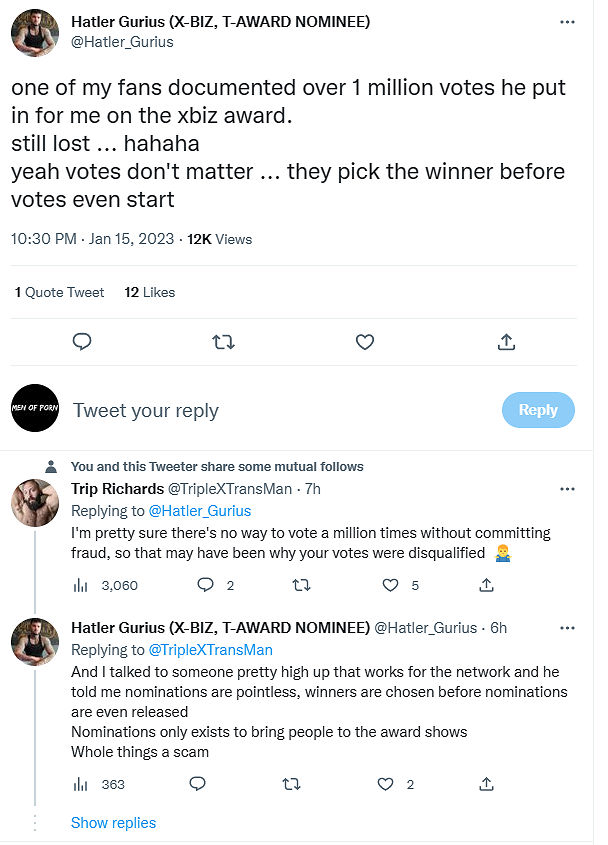**Detailed Caption:**

At the top of the image, there's a post from Hattler Gurius, an xbiz award nominee. His Twitter handle is @Hattler_Gurius. The tweet reads: "One of my fans documented over 1 million votes he put in for me on the xbiz award. Still lost... Ha ha ha. Yeah, votes don't matter. They picked the winner before votes even start." This tweet was posted at 10:30 p.m. on January 15, 2023, and has 12,000 views, one quote tweet, and 12 likes. The profile picture shows Hattler Gurius in a black tank top, showing off his arms.

Below this tweet, there are the standard Twitter interaction buttons: the reply bubble, the retweet arrows, the heart for likes, and the share icon. There is also a button that says "Tweet your reply" along with a blue "Reply" button. 

Additionally, it is noted that the user replying shares some mutual followers with the author. 

In the thread, there is a reply from Trip Richards (@TripleXTransMan) posted seven hours later, stating: "I'm pretty sure there's no way to vote a million times without committing fraud. So that may have been why your votes were disqualified." This reply includes a hands-raised emoji.

Hattler Gurius responded to Trip Richards, saying: "I talked to someone pretty high up that works for the network, and he told me nominations are pointless. Winners are chosen before nominations are even released. Nominations only exist to bring people to the award show. The whole thing's a scam."